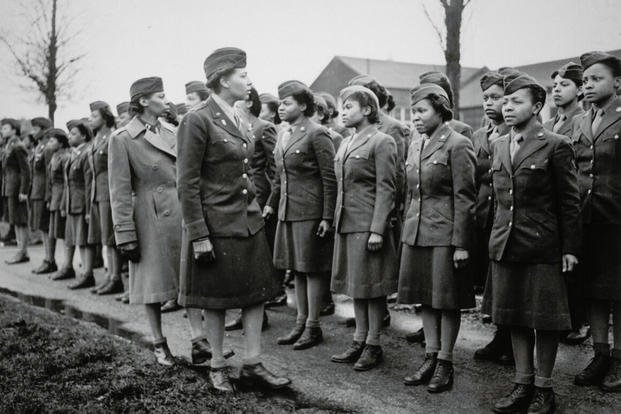This photo captures a historic black-and-white image from World War II featuring the distinguished 6888th Central Postal Directory Battalion, an all-Black, all-woman unit. The battalion members are standing at attention in three orderly rows, each woman clad in a standardized Army uniform that includes skirts, leggings, boots, and Army hats. The clarity of the image showcases their disciplined formation on a concrete surface, suggesting a daytime setting with bright lighting. A commanding woman, likely an officer, is seen inspecting the battalion, walking down the line in the same uniform. Accompanying her is another woman in a khaki trench coat and gloves, possibly her aide. The background reveals barracks and the tree trunks of two barren trees, emphasizing the outdoor setting devoid of foliage.